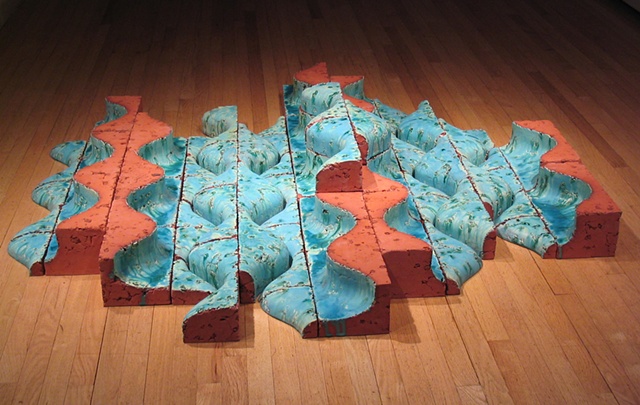The image displays an intriguing art installation set on a medium-toned, hardwood floor reminiscent of a basketball court. The installation itself consists of long, red clay bricks arranged in a staggered pattern. Each brick is meticulously carved to create wavy, melted-inset shapes, giving the impression of fluidity and movement. These wavy indentations are painted in gradient shades of light blue to turquoise, further enhancing the illusion of flowing water. The overall effect is an abstract, yet harmonious blend of textures and colors, juxtaposing the earthy red bricks against the cool, aquatic hues of blue, creating a visually captivating and thought-provoking piece.